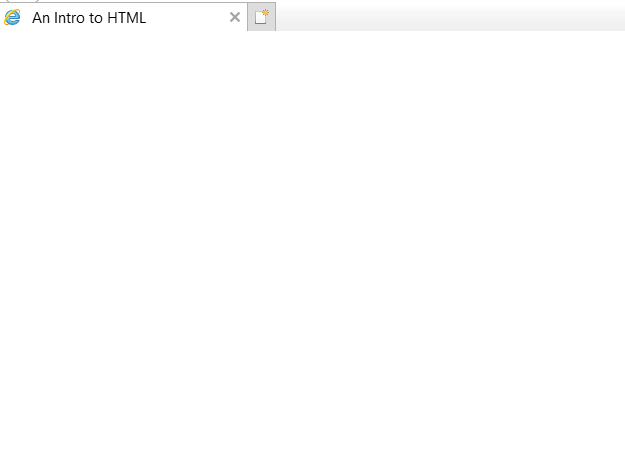The image appears to depict an incomplete or improperly loaded web page viewed in Internet Explorer. At the top of the page, there is the Internet Explorer logo. The only text visible on the page reads "An Intro to HTML," likely indicating the title or header of the intended content. To the right of this text, there is a small icon resembling a picture in a file folder with a gold star in the top right-hand corner; this might be a placeholder for an image or an icon that did not load correctly. Additionally, there is a faint, shadowy line running horizontally across the top of the page. Except for these details, the rest of the page is blank, suggesting a failed loading or rendering issue.